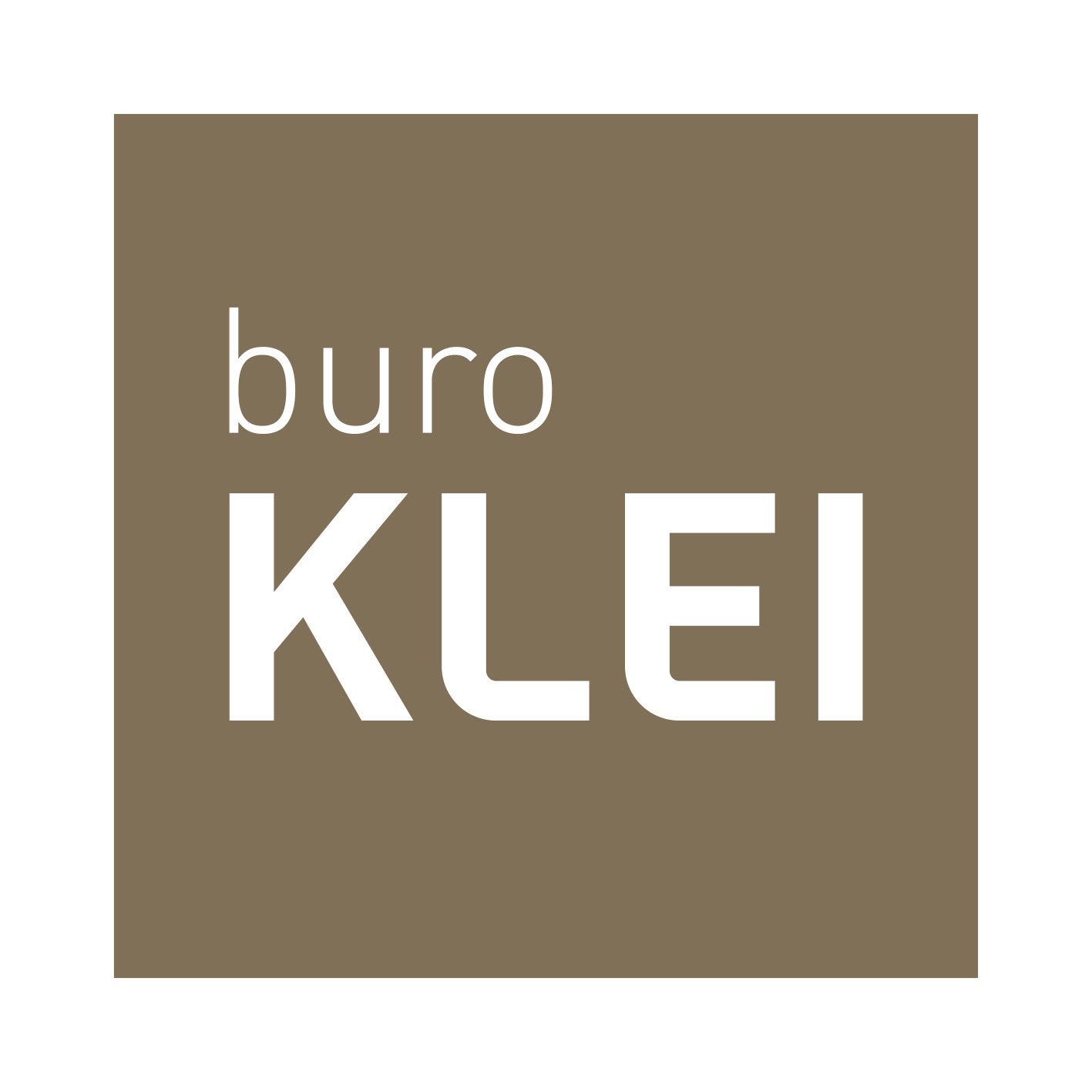The image is a computerized graphic that serves as a simple advertisement or sign. It is a square shape with dimensions approximately 4x4 inches, featuring a light brown, taupe background that falls between dark brown and beige tones. Centrally positioned are two sets of white text. At the top, in small lowercase letters, is the word "B-U-R-O." Below it, in a much larger and thicker capitalized font, is the word "K-L-E-I." Both sets of text have a unified white color and exhibit a slight rounded edge. The layout ensures "B-U-R-O" occupies the upper half while "K-L-E-I" dominantly fills the lower half, with no other elements, objects, or variations in color present in the image.